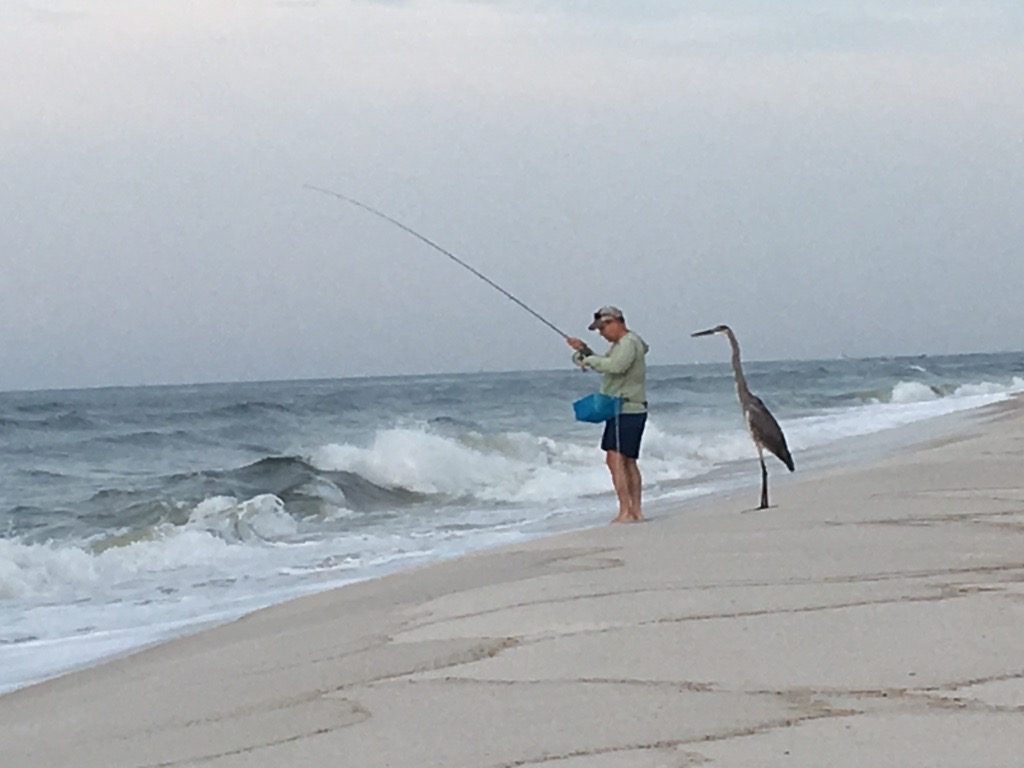In this color image, a man is fishing at the water's edge on a slightly overcast beach. The bottom 30% of the scene is covered in a brown tan sand, while the top 70% is dominated by blue, white, and gray ocean waves cascading towards the shore. The sky is misty gray blue, adding to the serene yet somewhat moody atmosphere. Centered in the image is a white man dressed in a tan hoodie and blue shorts. Barefoot, he holds a blue bucket in his left hand and a fishing rod extending over the water in his right. He appears focused, looking down at his hands. Notably, a tall, gray stork-like bird stands directly behind him, almost as tall as the man himself. The bird, upright and leaning slightly towards him, seems keenly interested in the fishing activity, offering a humorous contrast as it watches the man's every move, perhaps eyeing the potential catch. The ocean waves are crashing in, suggesting that the tide has been up, and the sand bears visible tide marks. The man also sports a hat with sunglasses on top and has a blue tackle box or bait container tied around his waist, emphasizing his preparedness for fishing.